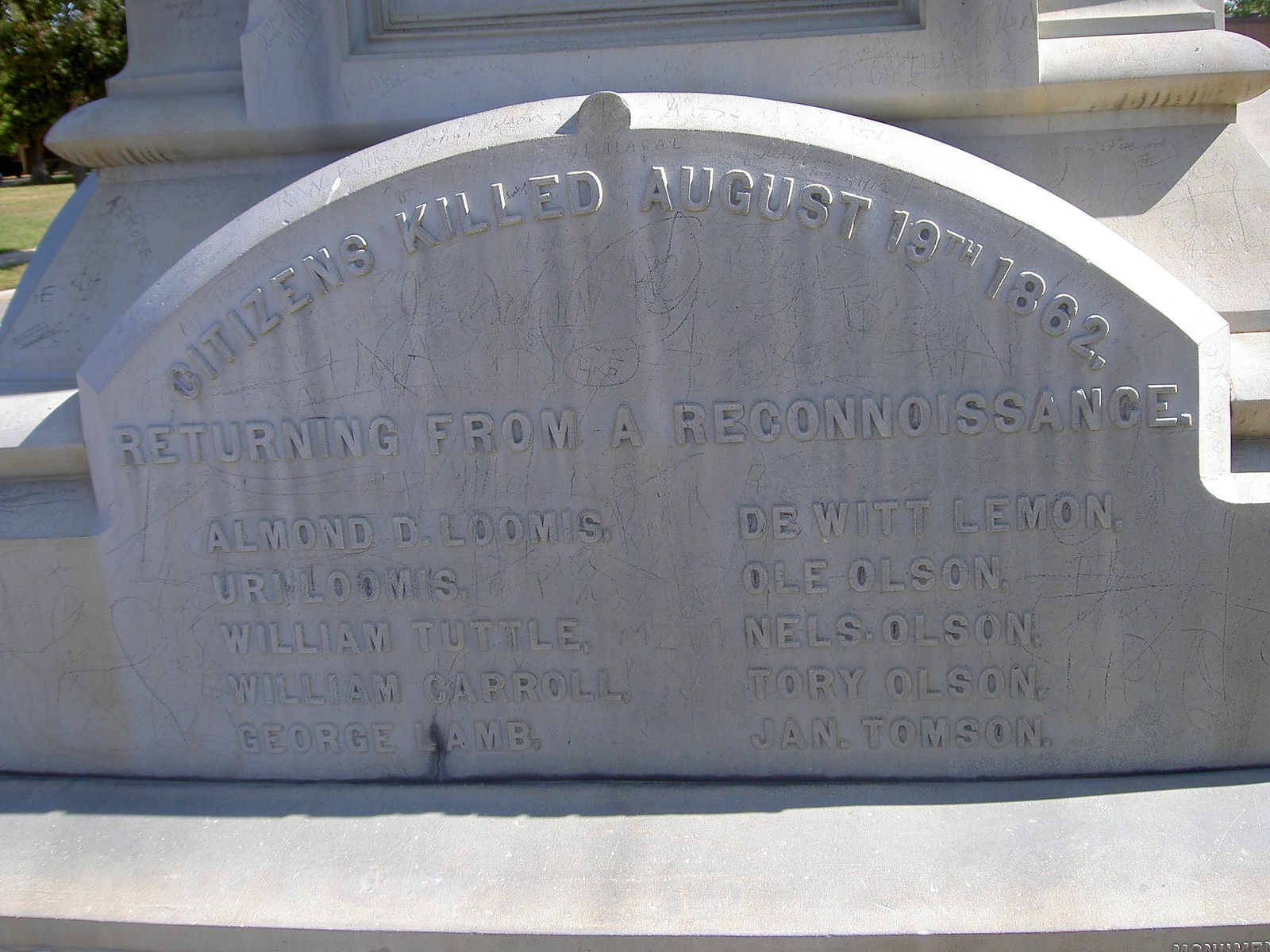The image depicts a beautifully large and detailed white arched memorial headstone, likely made of marble or granite, situated in a serene cemetery setting with green grass and trees in the background. The headstone is dedicated to commemorating "Citizens Killed, August 19th, 1862, Returning from a Reconnaissance." The names engraved in two columns include Armand D. Loomis, Uri Loomis, William Tuttle, William Carroll, George Lamb, DeWitt Lemon, Ola Olson, Nels Olson, Tori Olson, and Jan Thompson. Despite some black graffiti and scratches marring the surface of the stone, the engraved text remains clearly visible. Additionally, a larger monument with similar markings is visible in the background, and the sunlight softly illuminates the top of the memorial, enhancing the tranquility of the scene.